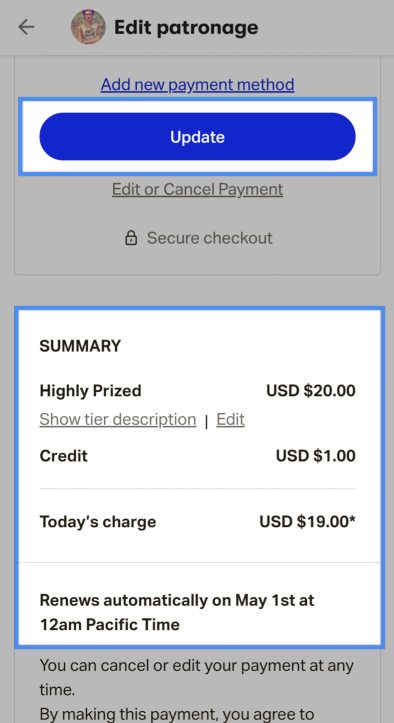The image features a white background page with a purple overlay, creating a two-layer effect. Text on the upper section of the purple page reads "Edit Patronage" in black, accompanied by an icon of a person. Below this, in blue text, it says "Add New Payment Method." 

In the foreground, a blue button with white text labeled "Update" stands out, outlined in a darker blue. Beneath this button, the background page displays additional text that states "Edit or Cancel Payment," followed by a lock icon and the phrase "Secure Checkout."

Towards the bottom, another section of the image is zoomed in, highlighting detailed information enclosed within a blue outline. This section contains the text "Summary," followed by "Highly Priced USD $20" and "Show Tier Description." Further down, it mentions "Credit $1," "Today's Charge $19," and specifies that the subscription will renew automatically on May 21st at 12 a.m. Pacific Time.

At the very bottom, there's a slightly obscured text indicating users can cancel or edit their payment at any time, along with a statement about agreeing to terms and conditions, which is partially cut off.